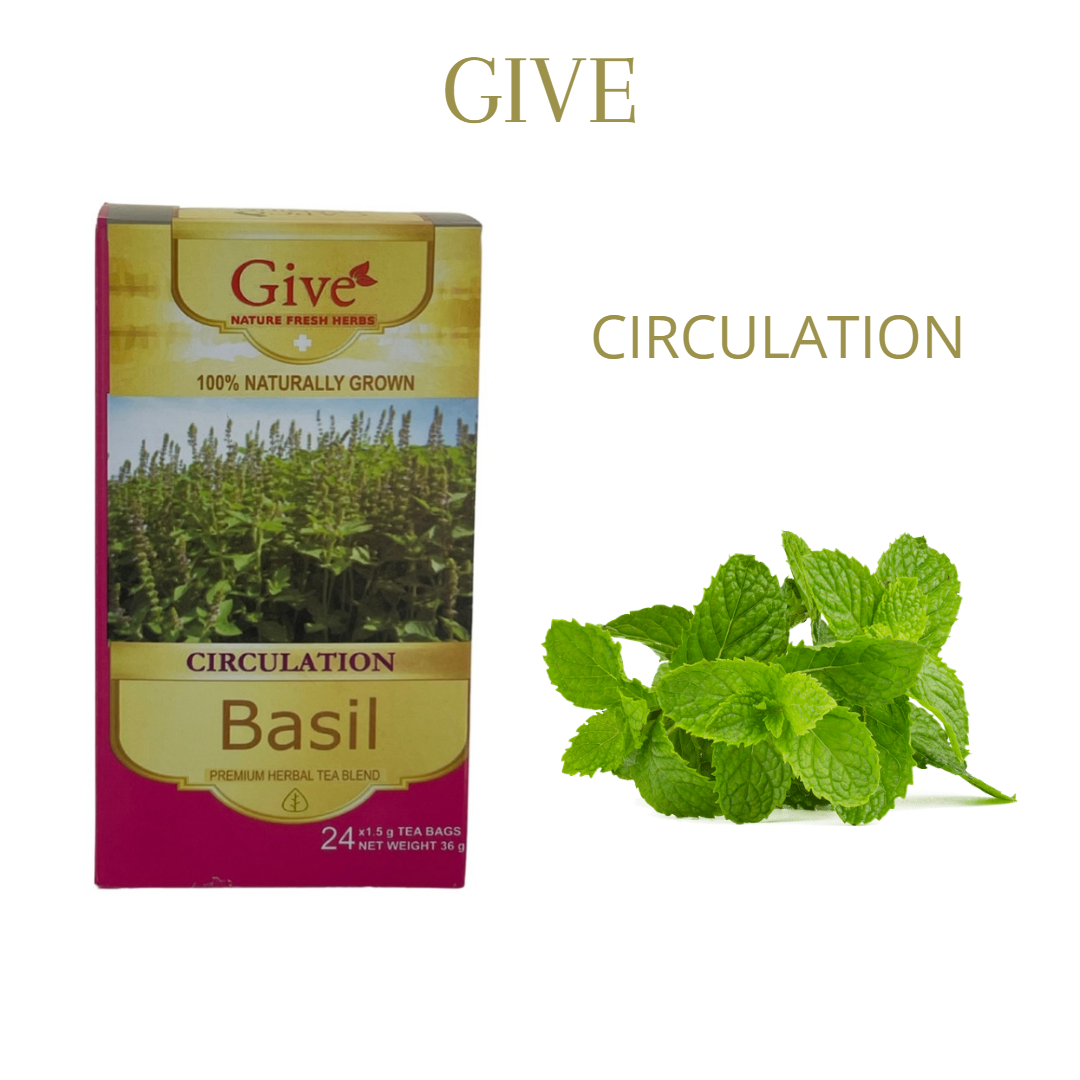The image is a detailed advertisement for a natural medicine, specifically a premium herbal tea blend made from basil. Featured prominently on the left side is the vertically-oriented package of the tea. The box has a striking reddish background with gold accents, including a wooden plaque-like design element at the top and a curved bumpy format at the bottom. The top part of the packaging reads "GIVE" in red with two small leaves over the "E," and "NATURE FRESH HERBS." Below this, a white medical plus icon is followed by the text "100% NATURALLY GROWN" in a dark brownish font. 

In the central portion of the box, there's a vibrant photographic image of a field of basil plants under a blue sky. Beneath this image, on the gold background, is the word "CIRCULATION" in purple, with "BASIL" in a goldish brown color under it. Further down, it says "PREMIUM HERBAL TEA BLEND," accompanied by a logo of a tea leaf. The bottom right corner details the contents: "24 x 1.5g tea bags, net weight 36g" in white text.

On the right side of the image, there are raw, fresh basil leaves resting on a pristine white background. Above these leaves, in gold-colored, all-caps text, the word "GIVE" is prominently displayed, followed by "CIRCULATION" in slightly smaller text. This thematic advertisement showcases the natural, health-focused benefits of the product through both text and imagery.